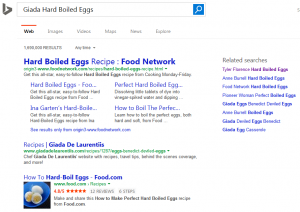This screenshot captures Bing search results for "Giada hard-boiled eggs". At the top left is the gray Bing logo, followed by a search box edged with a gray border and filled with a white background. To the search box's right is a blue square with a white magnifying glass icon. Below this is a navigation bar featuring six selectable tabs: "Web", "Images", "Videos", "Maps", "News", and an unreadable sixth tab. The "Web" tab is currently active, highlighted by a red line above it and bold black text, while the others are in gray text.

Directly beneath this bar, the first search result appears, titled in blue "Hard-Boiled Eggs Recipes - Food Network". Accompanying the title is a green URL and four sub-links arrayed in a 2x2 grid with no grid lines. These sub-links display titles in blue with subsequent descriptions in black text. The titles are truncated with ellipses: "Hard-Boiled Eggs FOO...", "Perfect Hard-Boiled Egg...", "Ina Garten's Hard-Boiled...", and "How to Boil the Perfect..."

Further down, there is a snippet from Giada De Laurentiis' recipe, marked by a green URL and a single-line description that extends into two additional words. Below this is another result from FOO.com which includes a thumbnail of a halved boiled egg in a blue bowl, showing the yolk. This entry also features user ratings represented by dark orange stars, averaging at 4.8.

On the right side of the screenshot, a column displays related searches. The first entry, "Tyler Francesco Hard-Boiled Eggs", is in purple, indicating prior selection. The remaining eight related searches are in blue and have yet to be clicked.